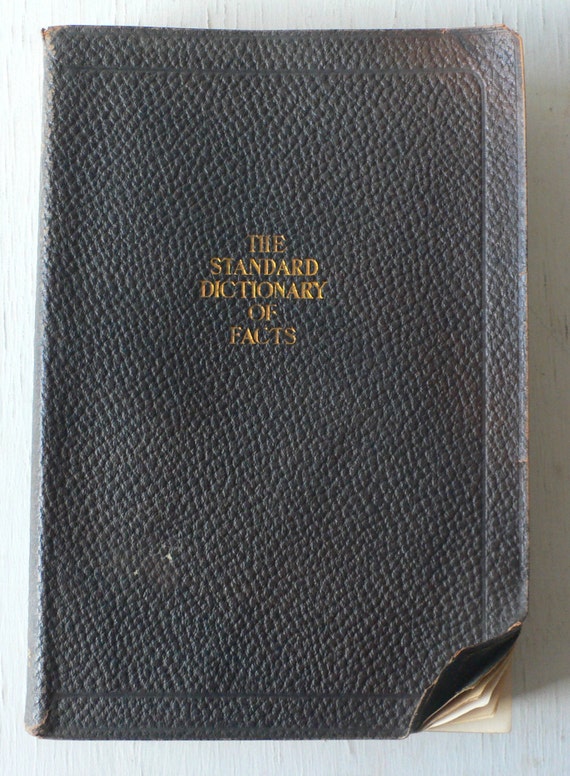The image depicts a vintage book titled "The Standard Dictionary of Facts," featuring a textured, black leather-bound cover with a line border near the edges. The title is prominently displayed in gold lettering in the center. The book shows significant wear, with the upper left corner of the cover damaged and some rubbing evident. In the bottom left corner, there is a small tear. The bottom right corner of the cover and several off-white, yellowed pages beneath it are folded upward. The book rests on a gray, textured surface. The details of the background are somewhat ambiguous, suggesting it might be a painted or wood surface with noticeable line textures, possibly indicating age. The binding reflects light, hinting at a light source coming from the left side.